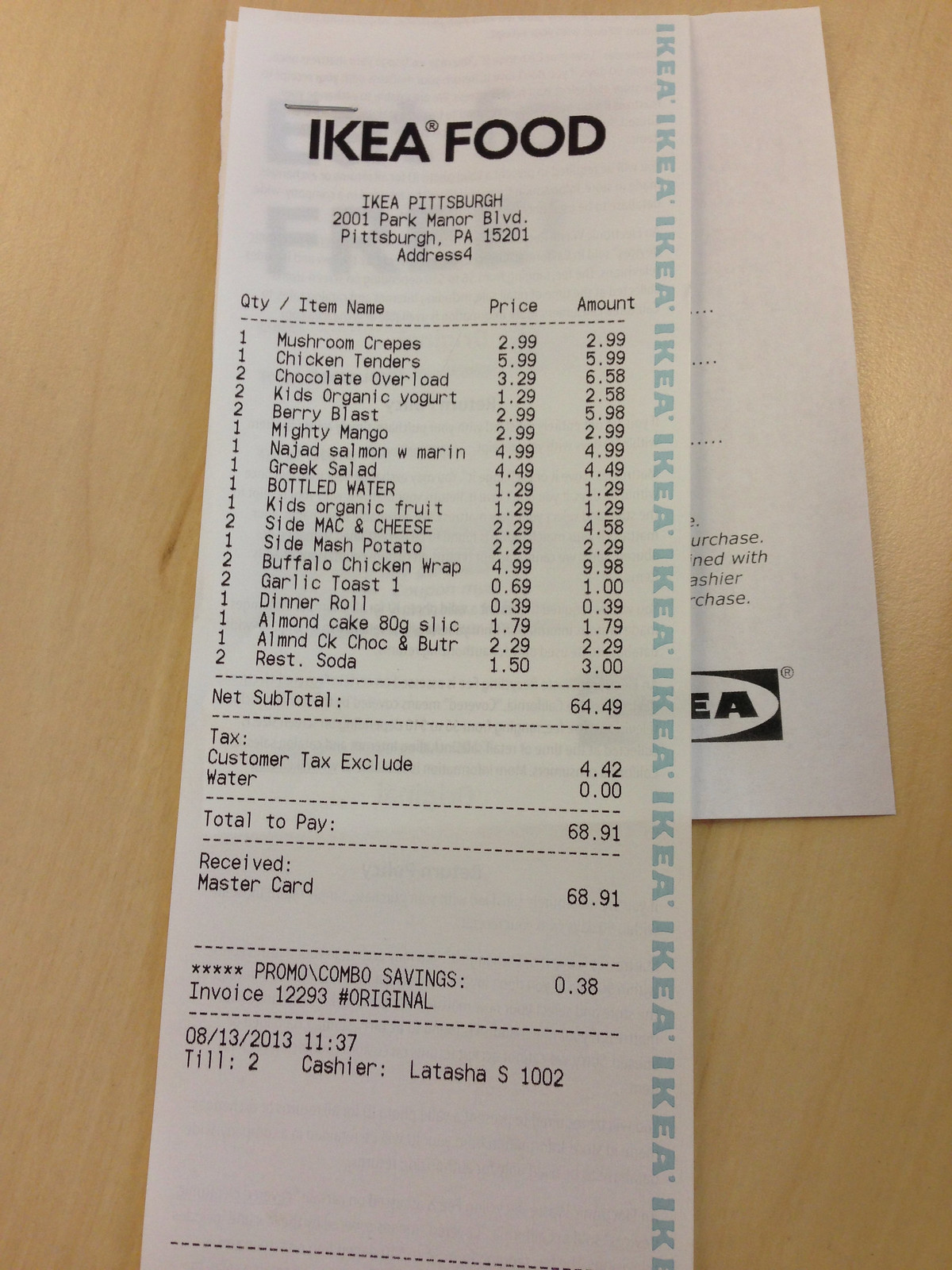This detailed close-up photograph captures a register receipt placed on a light brown wooden table, likely untreated plywood. The receipt, printed on traditional register paper in small black text, prominently displays "IKEA Food" at the top, indicating purchases made at the IKEA Pittsburgh restaurant located at 2001 Park Manor Boulevard, Pittsburgh, PA, 15201. The receipt meticulously lists various food items including:

- One Mushroom Cake ($2.99)
- One Chicken Tenders ($5.99)
- Two Chocolate Overload ($3.29 each)
- Two Kids Organic Yogurt ($1.29 each)
- Two Berry Blasts ($2.99 each)
- One Mighty Mango ($2.99)
- One Najad Salmon with Marron ($2.99)
- One Greek Salad ($4.49)
- One Bottled Water ($1.29)
- One Kids Organic Fruit ($1.29)
- Two Side Mac and Cheese ($2.29 each)
- One Side Potato ($2.29)
- Two Buffalo Chicken Wraps ($4.99 each)
- Two Garlic Toasts ($1.69 each)
- One Dinner Roll ($0.39)
- One Almond Cake, 80g slice ($1.79)
- One Almond Chocolate Butter ($2.29)
- Two Rest Sodas ($1.50 each)

The net subtotal is $64.49, with an additional customer tax excluded at $4.42, bringing the grand total to $68.91. The transaction was completed using MasterCard. This receipt, bearing invoice number 1.2293 and noted as the original copy, is dated August 13, 2013, at 11:37 AM, with Latasha S. serving as the cashier (register 1002). The light blue text down the receipt repetitively reads "IKEA."